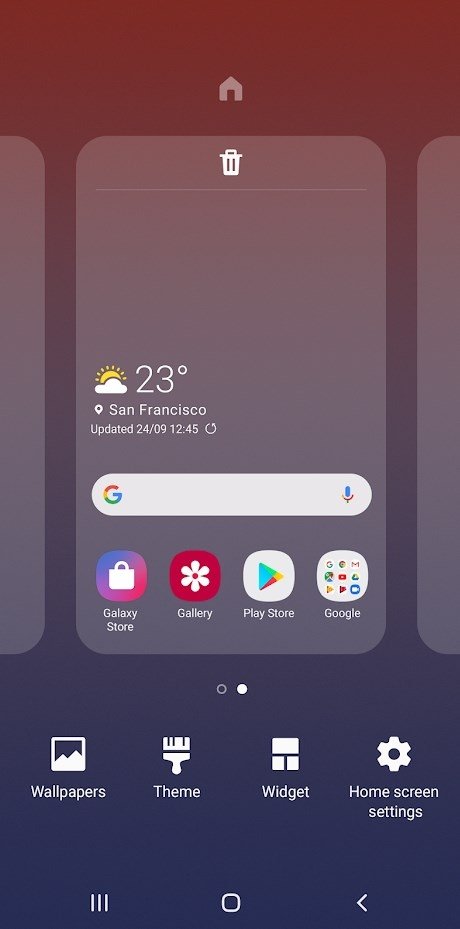The image depicts a person editing the home screen on a Samsung Android phone. The screen displays a vibrant background that transitions smoothly from a hazy blue at the top to a dark reddish-maroon hue at the bottom. The device's navigation bar at the bottom of the screen features three distinct icons: three horizontal lines, a square, and a left-pointing arrow, characteristic of Samsung's interface.

At the top of the screen, a transparent gray home icon is visible. Below it, there is a panel containing a Google Search bar and four app icons: Galaxy Store, Gallery, Play Store, and a folder filled with various Google Apps, identifiable by their colorful icons.

Additionally, a weather widget indicates that it is 23 degrees in San Francisco and partly cloudy, with a last update timestamp of 12:45. A reload icon accompanies this information.

The screen appears to be in a zoomed-out edit mode, with a small trash icon present for deleting the entire home screen. Towards the bottom, there are four editing options, each represented by distinct icons in white: Wallpapers, Theme (with a paintbrush icon), Widgets (three squares icon), and Home Screen Settings (gear icon).